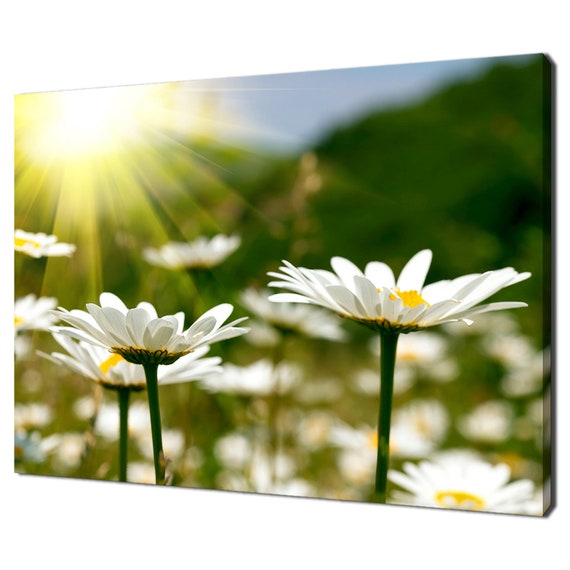The image is a vivid painting of wildflowers, resembling white daisies, with prominent green stems, white petals, and vibrant yellow centers. The composition is enriched by a bright, beaming sun in the upper left corner, casting radiant rays across the scene. In the foreground, a few flowers are sharply detailed, while numerous others fade into a blurred, lush green backdrop, suggestive of foliage or trees. The vantage point captures the scene at an angle, enhancing the illusion of depth as the left side appears smaller than the right, further emphasized by the 3D board display format. This tranquil, nature-inspired piece exudes peace, depicting the flowers stretching gracefully towards the sunlight, making it an ideal candidate to brighten any room with its serene beauty and vibrant depiction of a perfect weather day.